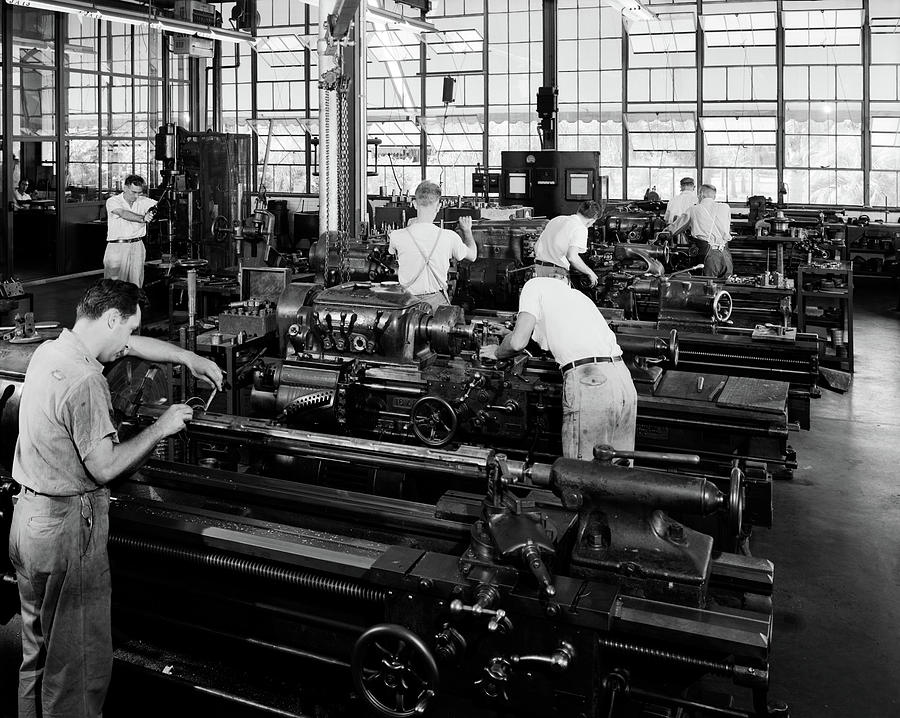This black-and-white photograph captures the bustling interior of a machine shop during the daytime. The setting features a row of rectangular metal tables equipped with pistons, gear dials, and wheels, each being serviced by various workers. Most of the men in the image are wearing white shirts and a mix of gray and white pants, many of them dirty from their labor-intensive tasks. 

In the left foreground, a white man with a set of keys hanging from his belt loop is adjusting a piston on the first piece of equipment. Ahead of him, another man wearing dirty white pants and a clean white t-shirt bends over the second table. Further into the scene, one man, distinguished by his apron and white shirt, holds onto a part of the equipment with a focused demeanor, while another man in gray pants and a white shirt with a black belt works intently on yet another table. Some of the men appear to be in profile, with their backs turned to the camera, adding to the sense of depth and activity.

In the background stands a large, open glass wall, flooding the workspace with natural light, supplemented by overhead fluorescent lights. To the left, a pillar with a chain and, beyond it, a man in black pants and a white shirt operates a different piece of upright machinery, possibly a stamping or dye tool. The space is filled with an array of industrial equipment, and the atmosphere is one of diligent work and mechanical precision. The photograph offers a detailed glimpse into the daily operations of a machine shop, populated by workers deeply engaged in their respective tasks.